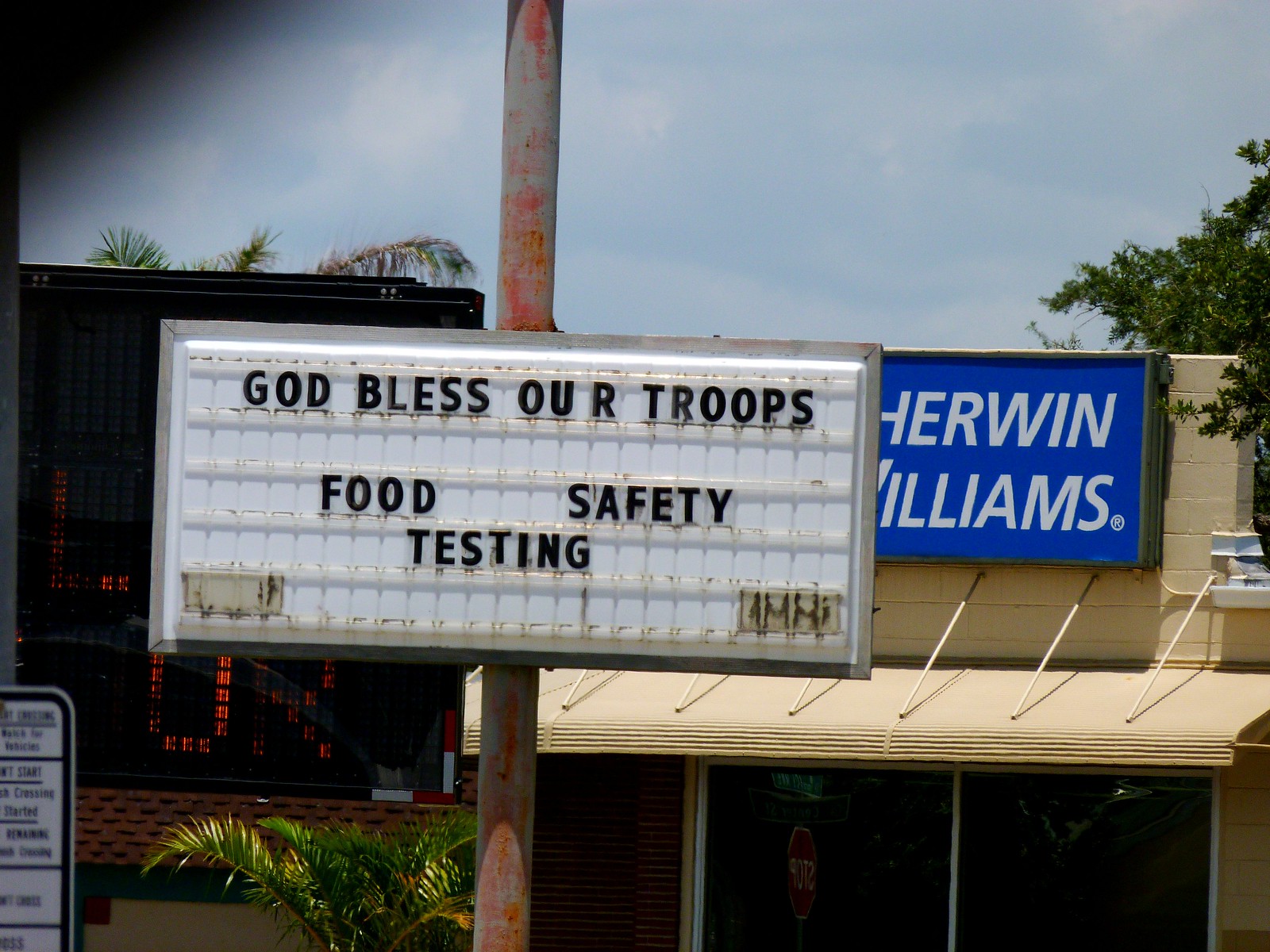A weathered marquee sign stands tall on a rusted pole, prominently featuring the black-lettered messages "God Bless Our Troops" followed by a separate line that reads "food safety testing." The sign is positioned in front of a one-story commercial building constructed from cinder blocks and bathed in the dim light of dusk. This building, branded with the Sherwin-Williams logo, indicates it is a paint store. The store's awning partially obscures the structure, beneath which a series of darkened windows hint at the interior but reveal nothing. The peculiar juxtaposition of the heartfelt patriotic sentiment and the mundane assurance of food safety on the marquee adds an element of unintended humor, likely prompting the photograph capturing this unconventional scene.